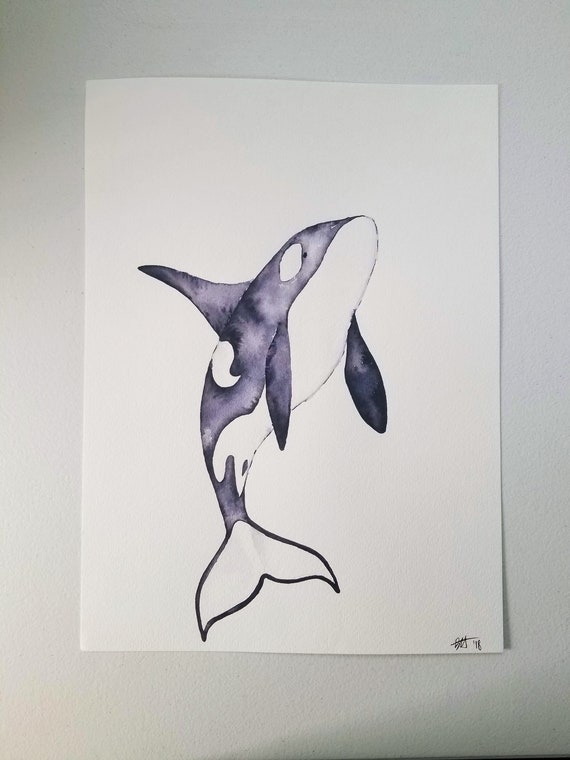This photograph captures an illustration of an orca whale executed in watercolor. The artwork, done on textured white paper, appears mounted or hung on a gray-textured wall, with its placement suggesting it is center-framed in the image. The watercolor painting features a whale depicted in hues of black with a purplish tint, contrasting against its white underbelly. Notable is the splotchy watercolored effect, especially in the darker areas. The orca is oriented vertically with its tail at the bottom of the paper and nose pointed upwards, and its two front fins angled downward. Additionally, the whale's tail is outlined in a darker black for emphasis. The white paper, likely 8 by 10 inches, is affixed to a larger backing, possibly with tape or glue, indicated by a lifted bottom corner. The image also includes a signature at the lower right, partially obscured but marked with the year '18, suggesting the work was created in 2018.